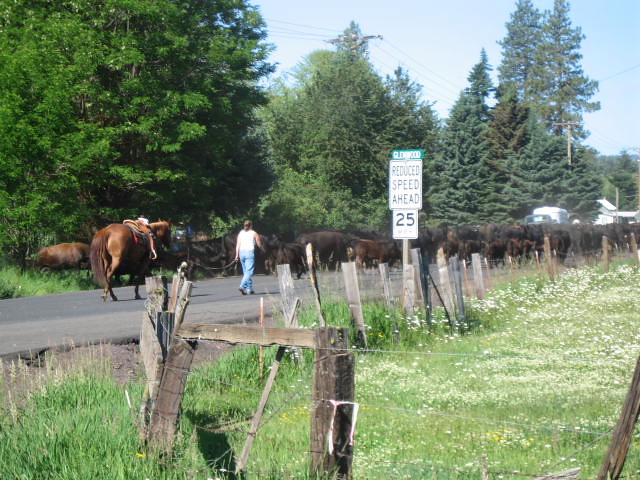In a bright, sunlit country setting, the photograph captures a woman walking away from the camera on a paved road with a lead in her hand, guiding a light-brown chestnut horse adorned with a saddle. The woman, wearing blue jeans and a white t-shirt with her hair pulled back in a ponytail, is accompanied by a large herd of predominantly dark-colored cattle further down the road. The road, emerging from the left side of the image, is flanked by green grassy fields and a somewhat dilapidated post and wire mesh fence. A "Reduce Speed Ahead" road sign, with the number 25 and additional unclear black writing, is prominently displayed near the fence on the right.

The backdrop features a diverse line of trees, including tall evergreens and leafy canopies, lending a vibrant mix of greens to the scene. Towards the right background, a vehicle and some buildings are faintly visible. The sky above is a strikingly clear blue, with few minimally visible clouds, completing the picturesque rural atmosphere.